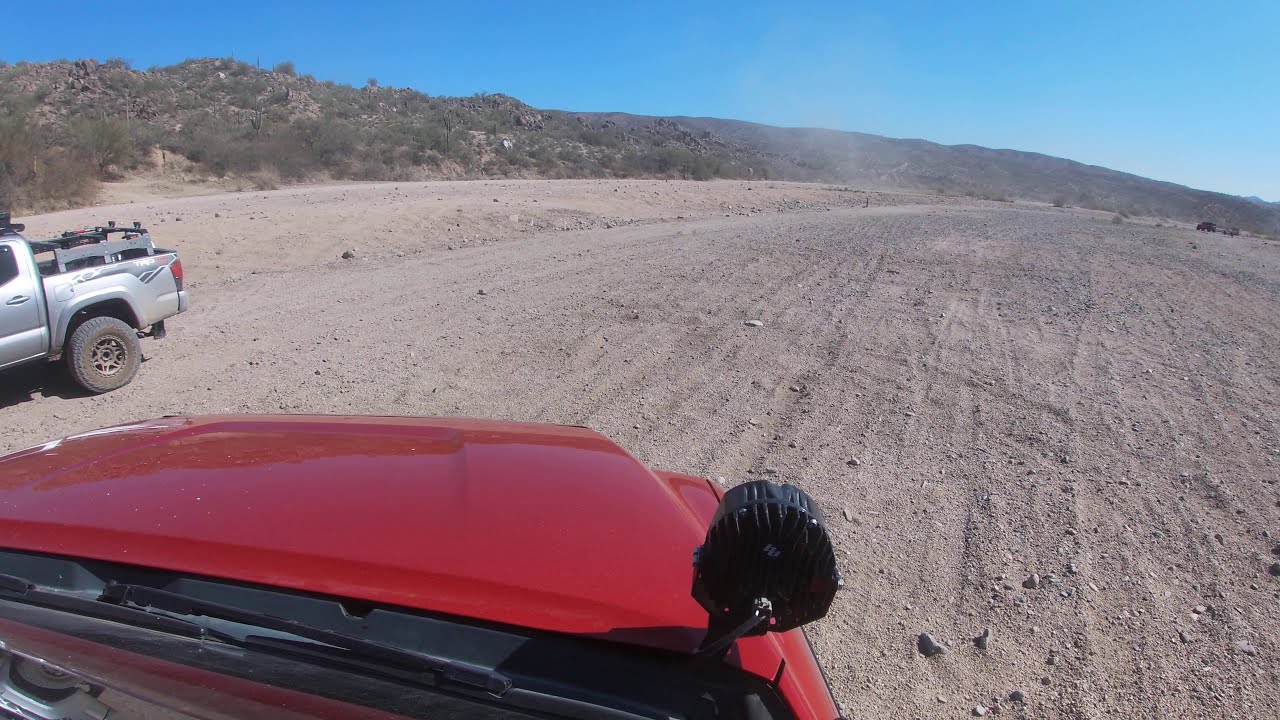This wide rectangular photograph captures a scenic off-road adventure from the perspective of the front seat of a red SUV. The bottom left corner prominently features the shiny, bright red hood of the vehicle, complete with a black windshield and a spotlight on the right-hand side. To the left of the SUV, the silver back half of a pickup truck—possibly a 4Runner—can be seen, equipped with a large black air intake on the hood, indicative of its off-road capabilities.

The dirt road, a light sandy path peppered with small gray rocks, stretches upwards towards the horizon where it curves and disappears. Just visible in the upper right corner are two small vehicles in the distance, adding to the sense of a vast, open space. The horizon line is marked by a lush green hill, sprinkled with trees and bushes, standing in stark contrast to the gray-brown gravel road. Topping off the scene is a perfectly clear, cloudless blue sky, suggesting a beautiful, sunny day ideal for off-road exploration.